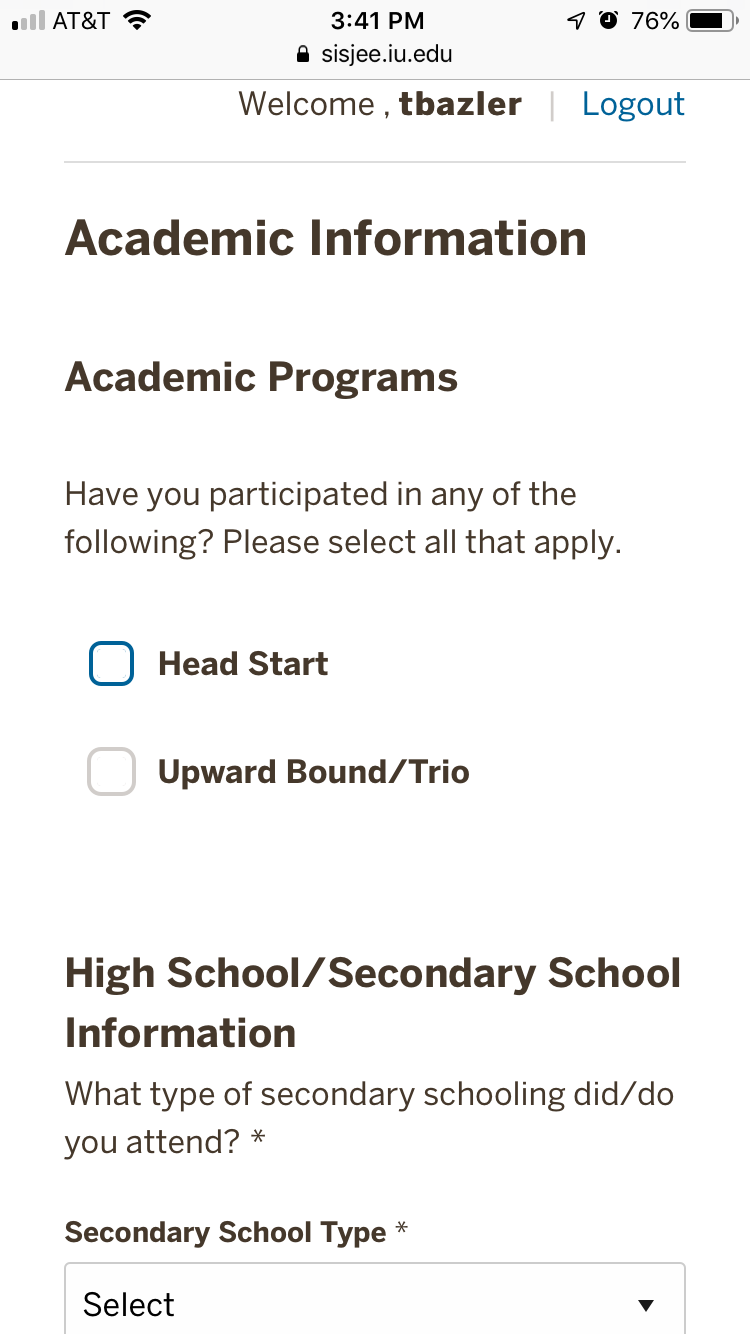A user is interacting with their phone on an academic website, specifically the Student Information System at Illinois University (sisjee.iu.edu). The webpage displays a welcome message for T. Basler, with a logout button next to their name. The site includes sections for academic information and programs, prompting the user with questions such as participation in programs like Head Start or TRIO/Upward Bound, with options to check any that apply. As they scroll further, they encounter a section titled "High School/Secondary School Information" where they are required to select the type of secondary school attended from a dropdown menu. The form appears to pertain to an application process, characterized by a clean white background and black text.